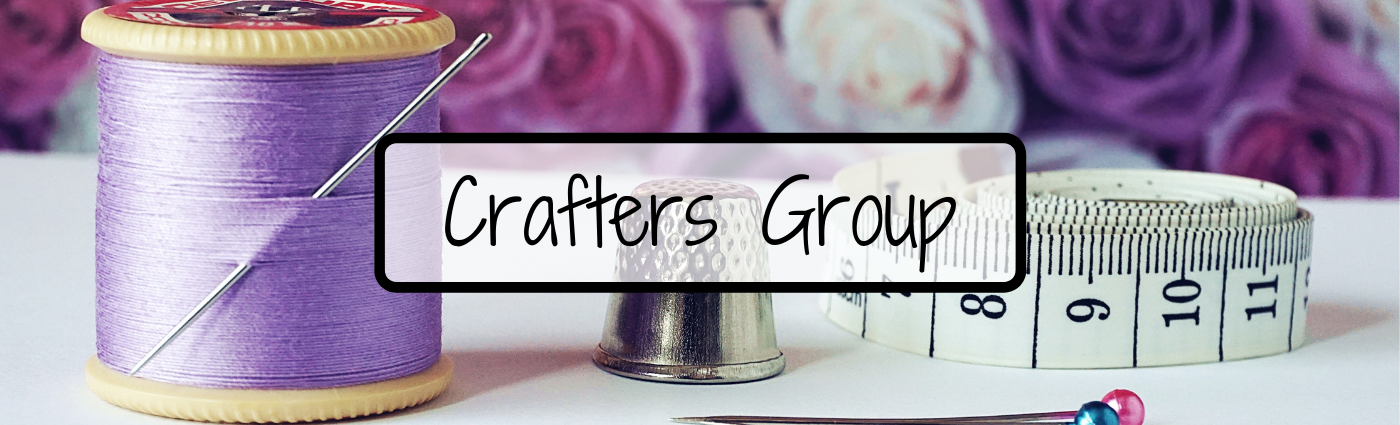This vibrant, full-color photograph captures a carefully arranged sewing scene against a backdrop of lush, blooming roses in purple, pink and white hues. Central to the arrangement, a banner with a black border prominently displays the words "Crafters Group" on a white background. To the far left, a gold-colored spool of purple thread stands upright with a needle poking through it at a diagonal angle. Positioned beside the spool is a silver thimble adorned with indentations on its top. Next to the thimble lies a white measuring tape marked with black numbers and lines for precise measurements. At the bottom of the picture, two straight pins rest on a pristine white table; one pin is tipped with blue and the other with pink. This horizontal rectangle image vividly showcases essential sewing tools framed by a delightful floral background, encapsulating the essence of a crafter's workspace.